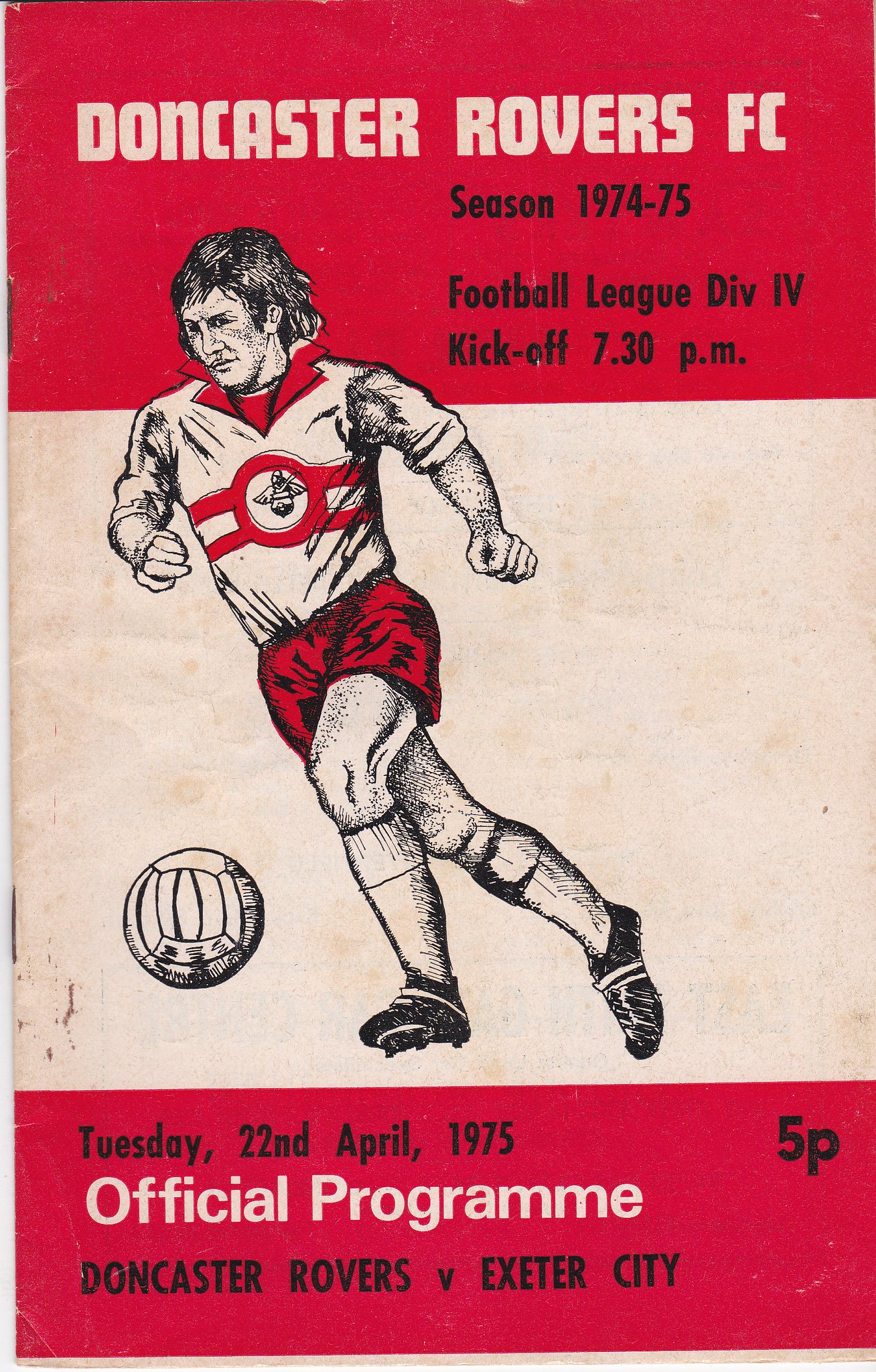The cover of a football program for Doncaster Rovers FC is set against a dark red background, with "Doncaster Rovers FC" prominently displayed at the top in white text within a light red bar. The season "1974-75 Football League Division 4" and the kickoff time "7:30 p.m." are inscribed in black. Below this header, a cartoonish illustration of a footballer, dressed in knee-high white socks, black cleats, red shorts, and a red-collared white polo featuring a circular red emblem, is depicted kicking a ball. The information continues beneath the illustration, stating "Tuesday, 22nd April 1975" in black text, with "Official Program" in white. Another line reads "Doncaster Rovers vs Exeter City," followed by the price "5p" on the right side.